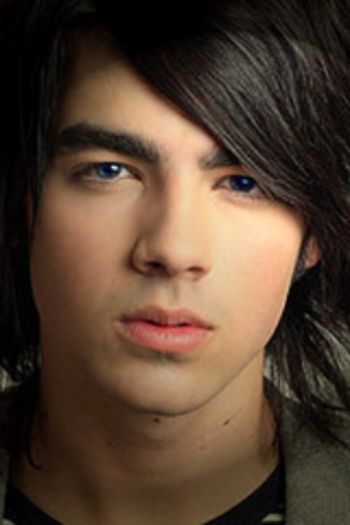The image features a close-up shot of a young man with blue eyes and olive skin, displaying a serious, pouty expression as he looks directly at the camera. His thick, black hair has an emo hairstyle, with bangs covering a large portion of his forehead and partly veiling his left eye. His eyebrows are dark and heavy. He is clean-shaven, and on his neck, a few small moles or freckles are visible. He is wearing what appears to be a black t-shirt, possibly with some white areas or stripes, and a jacket that seems to be either gray or brown. The photograph captures him from the top of his head down to just below his neck, including a small portion of his left shoulder. His face, neck, and hair occupy the majority of the image, suggesting he might resemble one of the Jonas Brothers.